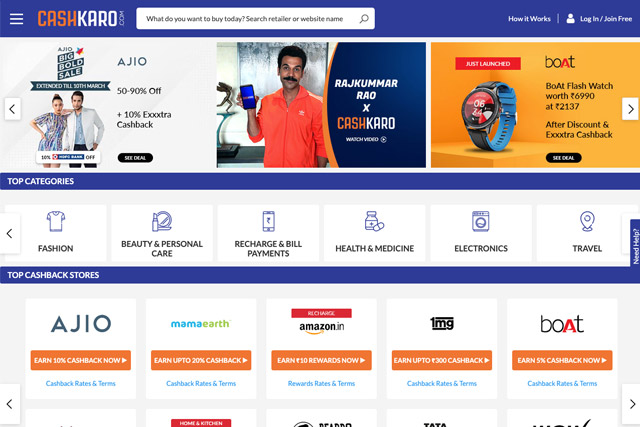The website boasts a vibrant and colorful design, prominently featuring shades of yellow, orange, white, and blue, with blue being the dominant hue. In the top left corner, there's a compact menu, while to its right, the brand "Cash Coral" is showcased alongside its web address, cashcoral.com. Adjacent to the brand name is a search bar prompting visitors with, "What do you want to buy today?" Just beside the search bar lies a "How it works" section, with the top right corner offering "Login" or "Join Free" options.

The upper half of the site is occupied by a dynamic banner highlighting various brands and promotions. Notable mentions include AGIO with discounts ranging from 50% to 90%, and a "Big Bold Sale". A collaboration is also highlighted featuring Rajkummar Rao and Cash Coral. Furthermore, there is a spotlight on a newly launched product: the Boat Flash Watch, originally priced at 6,990 currency units, now available for 2,137 units post-discount.

Below the banner, the site categorizes major sections such as Fashion, Beauty & Personal Care, Recharge & Bill Payments, Health & Medicine, Electronics, and Travel. Featured prominently are the top cashback stores with their respective logos, including AGIO, Mama Earth, Amazon.in, 1MG, and Boat (B-O-A-T). Each logo is followed by an orange button labeled "Earn Cashback", encouraging users to take advantage of these offerings.